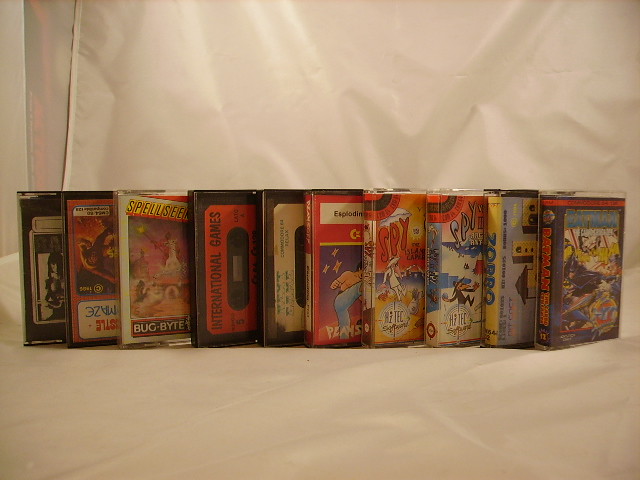This image showcases ten vintage media items that are likely old computer games or possibly cassette or VHS tapes, neatly arranged side by side on a white background or canvas. Among the recognizable titles are "Batman," "Spy vs. Spy," "International Games," "Spellseeker," "Pac-Man," and "Zorro." Each item is positioned upright, revealing their colorful and varied themes, which include comics and martial arts. There is also a notable item with the word "MAZE" visible at the bottom. The background is stark and white, enhancing the focus on these nostalgic pieces of media history.